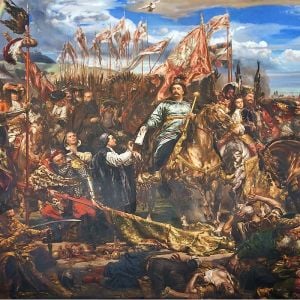A vibrant, busy painting captures the chaos of a battlefield scene under a blue sky with white clouds. The painting features numerous people, many of whom are carrying reddish-brown and white flags. Some figures are alive, engaging in activity, such as a central person on horseback who wears a light blue-gray or greenish-gray jacket, hat, and possibly a mustache. This central figure holds a golden staff and appears to be handing a piece of white paper to another person on the ground. The battlefield itself is littered with debris and bodies, strewn with flags and surrounded by wooden flagpoles. Other people can be seen standing and interacting, some wearing robes. The painting also includes several details like horses and their ornate trappings, adding depth to the chaotic yet meticulously detailed scene.